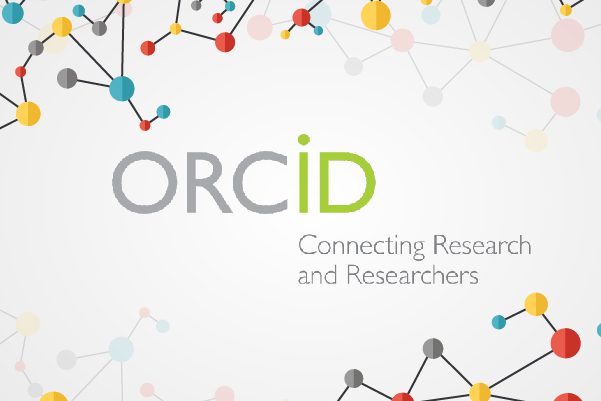The image depicts the homepage of a scientific research organization named ORCID. The organization's name is presented prominently, with the letters "O-R-C" in gray and "I-D" in lime green. All the letters are capitalized except for the "i," which, though lowercase, stands at the same height as the other letters, causing its dot to extend above the rest of the word.

The background of the page is a very pale gray. Below and to the right of the ORCID logo, the slogan "Connecting Research and Researchers" is displayed. The page is adorned with stylized, molecule-like graphic elements that surround the text. These elements consist of circles connected by black lines; the circles come in colors such as blue, pale blue, gray, yellow, and red. 

The molecule graphics are designed with shaded effects: each circle is divided down the middle, with the left half in a lighter shade and the right half in a darker shade of the same color. The elements in the upper left and lower right corners are rendered in full color, while those in the upper right and lower left corners are faded, adding a layered visual effect to the design.